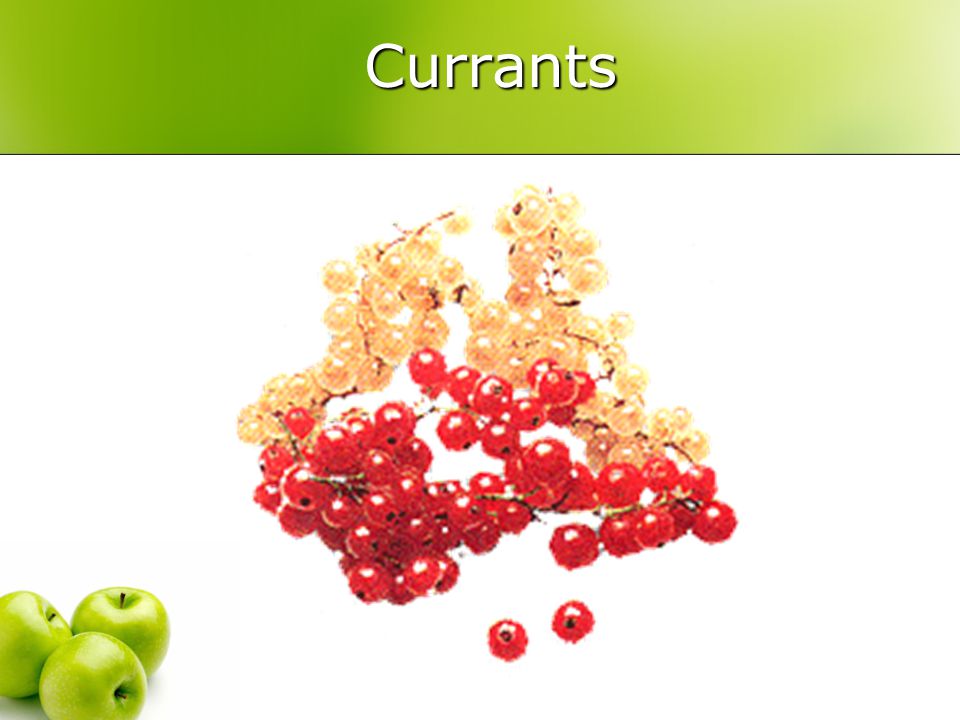The image features a white background and appears to be part of a fruit advertisement or presentation slide. At the top, a variegated green band (shading from dark on the left to light on the right) spans the upper center, emblazoned with the word "currants" in bold white letters. Centered beneath this text is a cluster of small, shiny berries on thin brown branches. The berries transition from a vibrant red at the center to a lighter golden color towards the top, depicting either ripeness stages or different varieties. In the lower left-hand corner, three flawless, vibrant green apples, likely Granny Smiths, are arranged – two laying on their sides and one standing upright, each with its black stem intact. The minimalist white background accentuates the colorful fruits, making them the focal point of the image.